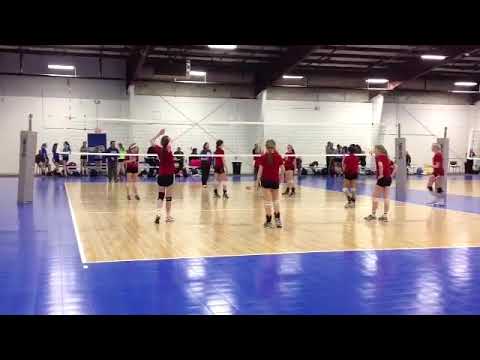In this detailed photographic image of an indoor volleyball match set in a gymnasium, the foreground prominently features four women dressed in red jerseys and black shorts, actively engaged in the game. Annette is positioned near the forefront, with opposing team members, also clad in red jerseys and black shorts, seen behind her. The scene is illuminated by a series of fluorescent lights installed above the court. The volleyball court itself is light brown, bordered distinctly by a blue boundary line.

The gymnasium’s white walls serve as the backdrop, against which a series of spectators, potentially including parents, other teams, and a coach, are gathered, observing the action. The ceiling and rafters are silver or gray, adding to the modern indoor aesthetic. Gray posts support a white volleyball net stretched across the court. The shiny wooden floor of the court reflects the overhead lights, enhancing the brightness of the scene. The entire setup suggests an intensely competitive environment, capturing the dynamic and energetic atmosphere of the volleyball match.